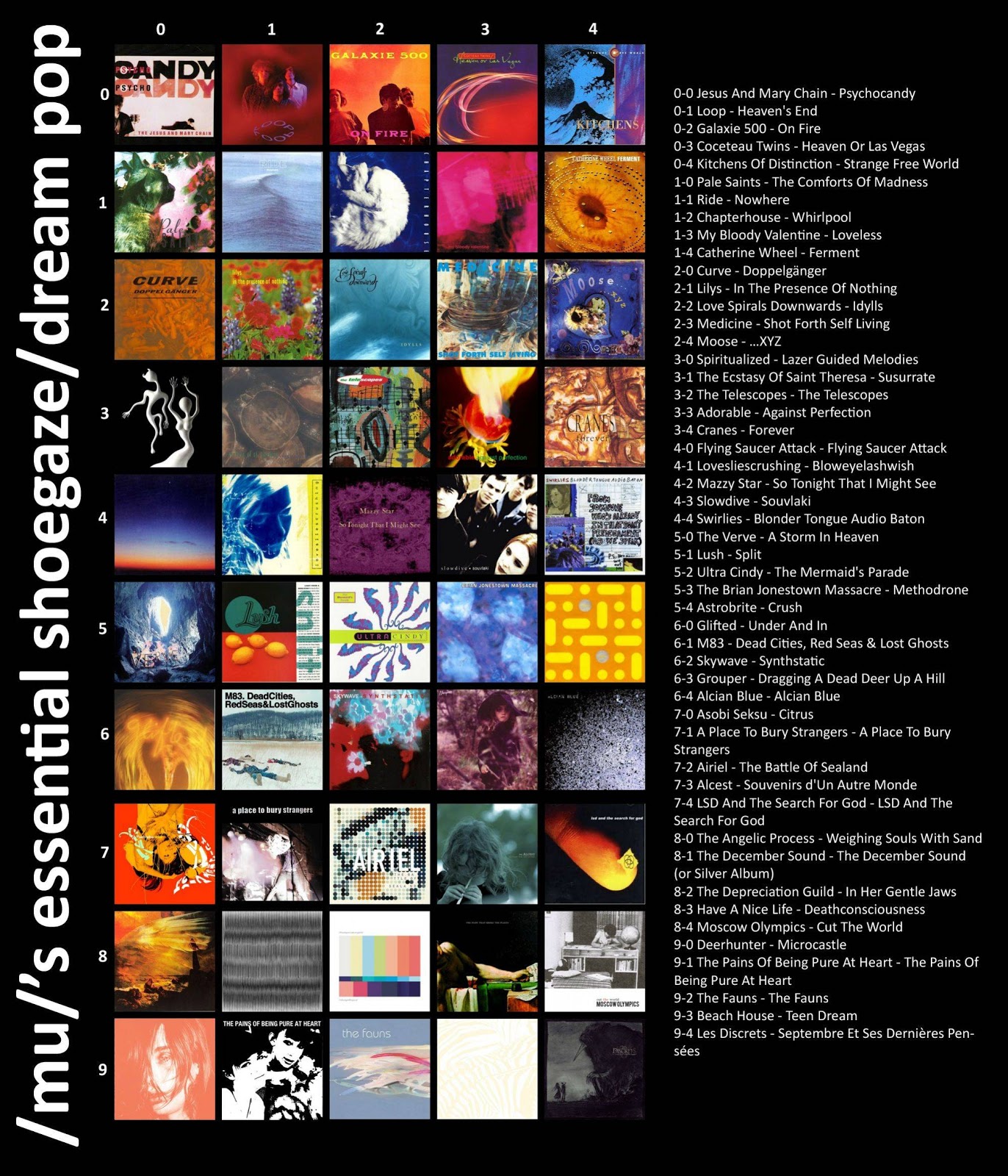This fan-made web page showcases the ethereal music genres of Shoegaze and Dream Pop. The site features a section titled "Muse: Essential Shoegaze/Dream Pop," which highlights influential bands and albums in these genres. On the left side, there's a collection of iconic album covers, while the right side lists essential tracks from notable bands. Some featured bands include Loop with their song "Heaven's End," Galaxie 500 with "On Fire," Lush with "Spooky," and The Verve with "A Storm in Heaven." Although some bands may be less recognizable, this curated selection represents the personal favorites and essential tracks according to the page's creator.